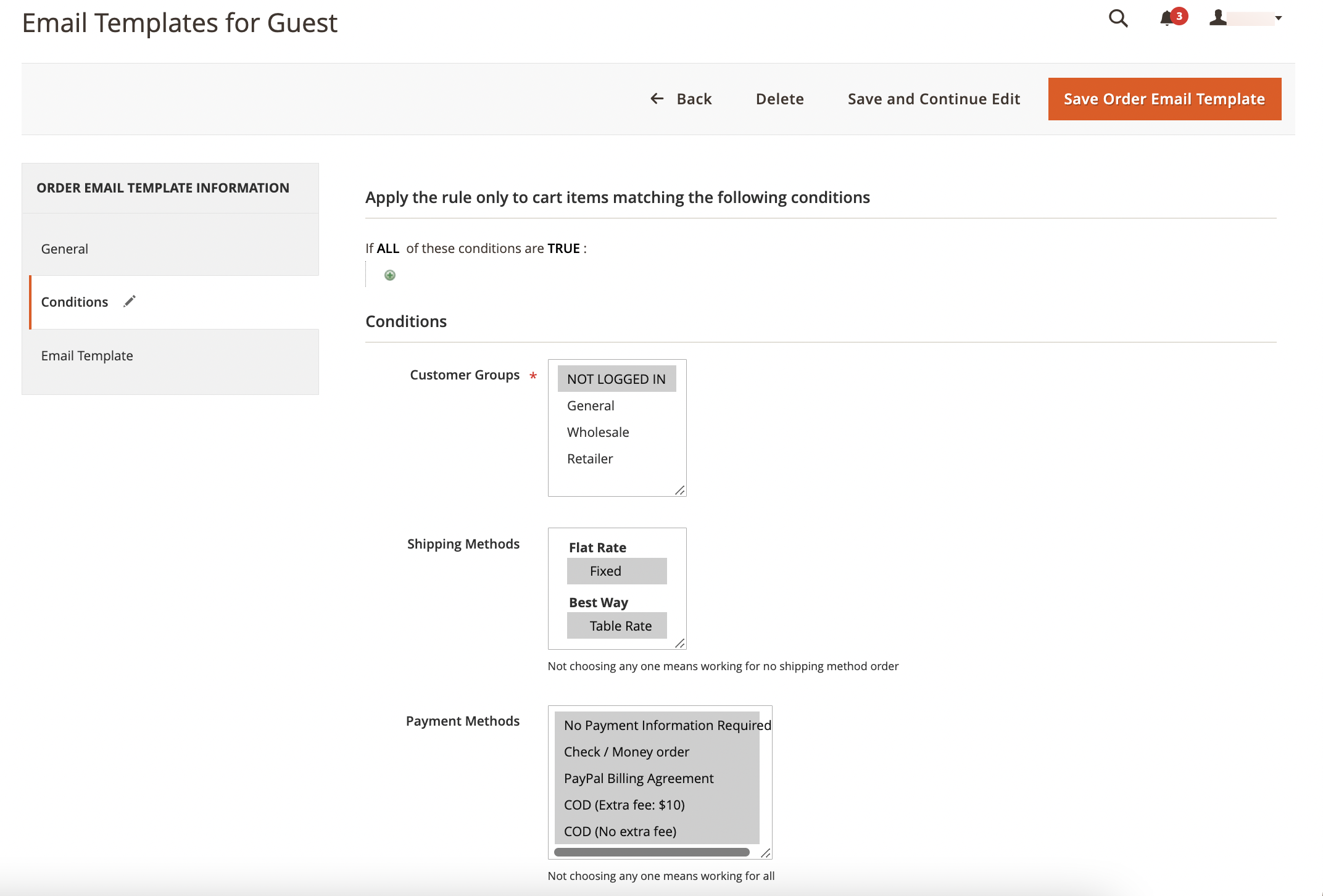In the image, the top left corner displays the words "Email Templates for Guests" in black text. On the top right, there is a profile icon of a person, flanked to the left by a bell icon with a number 1 inside a red circle, indicating a new notification, and further left by a magnifying glass icon, suggesting a search function. Centrally positioned at the top right are multiple textual elements: "Save Order Email Template" is prominently featured in white text on an orange rectangular background to the far right. To its left, the options "Save and Continue Edit," "Delete," and "Back" appear, with an arrow pointing to the left accompanying the "Back" option.

In the middle left of the image, a small square with a gray background is visible. At the top of this square, the words "Order Email Template Information" are displayed. Below this header, there are three tabs labeled "General," "Conditions," and "Email Template." The "Conditions" tab is highlighted with a horizontal white background and an orange vertical line on its left side. To the right of the "Conditions" tab, a small gray pencil icon signifies an edit function.